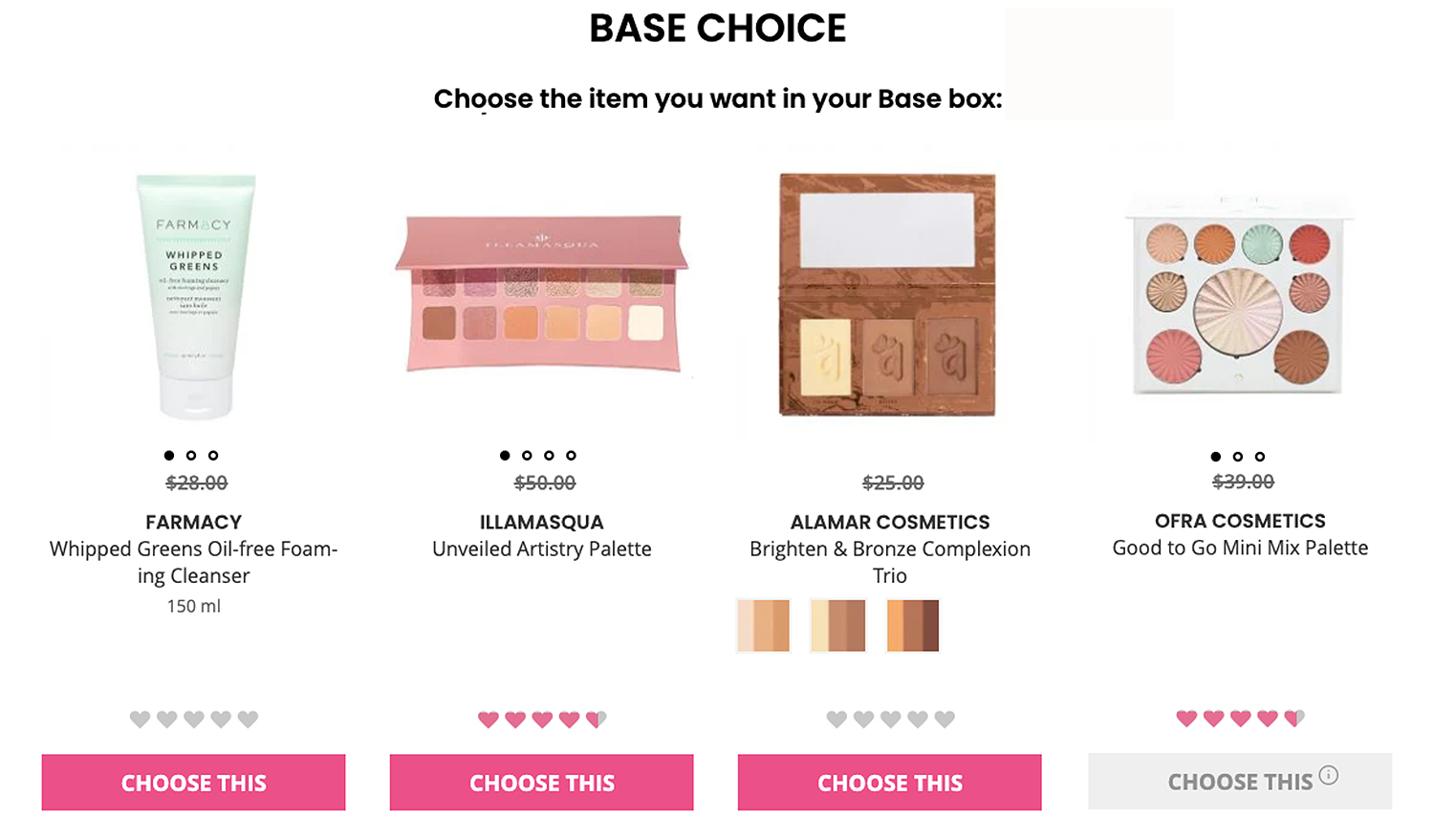The image features a white background with the heading "BASE CHOICE" in bold, black capital letters at the top. Below this, in smaller, non-capital letters, it reads "choose the item you want in your base box." 

On the left side, there's an image of a plastic tube labeled "Pharmacy Whipped Greens Oil-Free Foaming Cleanser, 150 milliliters." The original price of $28.00 is struck through, indicating a discount. Beneath the description, there is a prominent pink button labeled "choose this."

To the right, a pink container filled with various makeup products is displayed. This item is identified as the "Illamasqua Unveiled Artistry Palette" and is originally priced at $50.00, also struck through to show a discount. The product has a rating of four and a half stars, and below it, another pink "choose this" button is available.

Further to the right, a wooden item labeled "Alamar Cosmetics Brighten & Bronze Complexion Trio" is shown. The price of $25.99 is struck through, suggesting a discount. This product does not have a star rating or any hearts beside it. Below it, yet another pink button marked "choose this" invites selection.